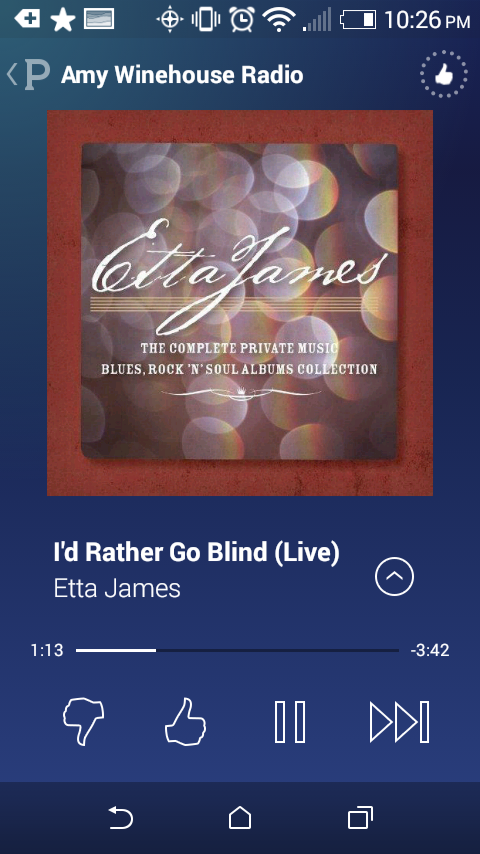This image is a detailed screenshot from the Pandora app on a mobile device. The central focus is Etta James's album "The Complete Private Music Blues Rock 'N' Roll Soul Albums Collection," specifically playing her song "I'd Rather Go Blind (Live)." The song is 1 minute and 13 seconds into its 3 minutes and 42 seconds duration. Displayed in a vibrant palette of red, gray, yellow, purple, and white, the album artwork contrasts against a blue background. At the top of the screen, typical mobile status icons like a clock showing 10:26 p.m., a nearly depleted battery indicator, and a Wi-Fi signal are visible. Below the album artwork, control buttons for thumbs up, thumbs down, pause, and skip are neatly arranged. Additional navigation icons for returning home and browsing are placed at the bottom. The text on the screen prominently reads "Amy Winehouse Radio," aligning with the overall setting of the Pandora app, and indicating the user's current station.